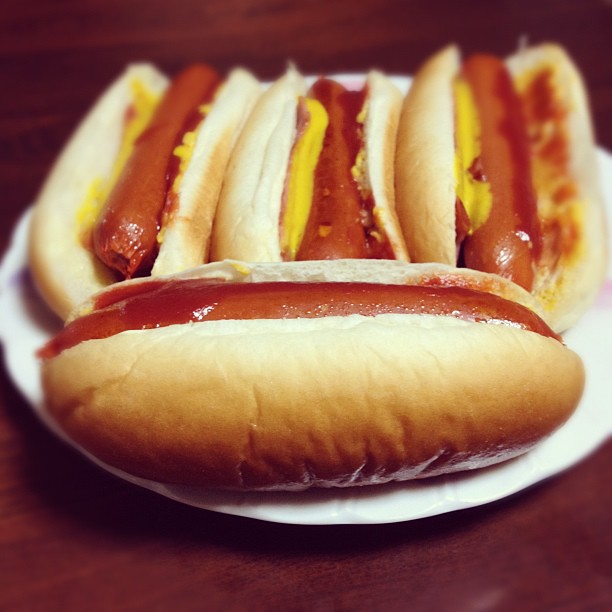This detailed photograph captures four hot dogs, each nestled in a golden-brown bun, arranged on a white, round plate. The plate, which appears to be ceramic, rests on a tabletop distinguished by its dark, mahogany stain and prominent wood grain. Three of the hot dogs are aligned vertically at the top of the plate, while the fourth hot dog is positioned horizontally at the bottom. Each hot dog is seasoned with a stripe of ketchup on one side and mustard on the other, though the bottom hot dog seems to only have ketchup, lacking the mustard typically found on the others. The hot dogs themselves are well-cooked, exhibiting a plumpness with beads of sweat hinting at their boiled preparation. Their golden brown-pinkish hue contrasts nicely with the white inner part of the buns.